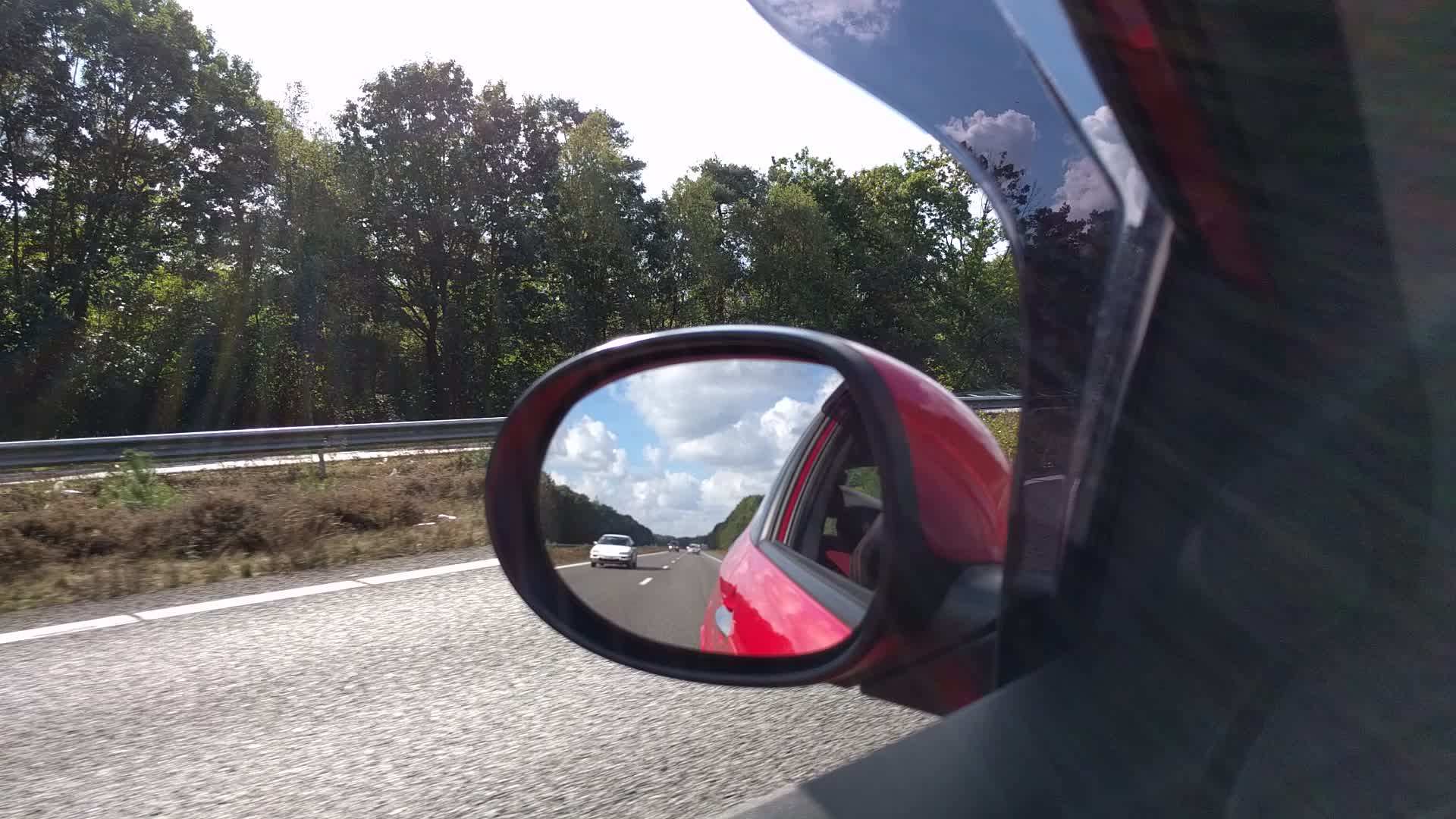The photograph captures a side-mounted rear-view mirror on the driver's side of a red car, taken from the perspective of an American driver while the vehicle is in motion. In the mirror's reflection, the road stretches behind, revealing a smooth, gray surface with a vivid blue sky overhead, adorned with white, fluffy clouds. A white car travels in the adjacent lane, trailing behind. The scene outside the mirror features a protective guardrail, a median strip, and a lush row of thick, green trees lining the roadside. The image beautifully blends elements of movement and tranquility, showcasing the dynamic yet serene journey on an open road.